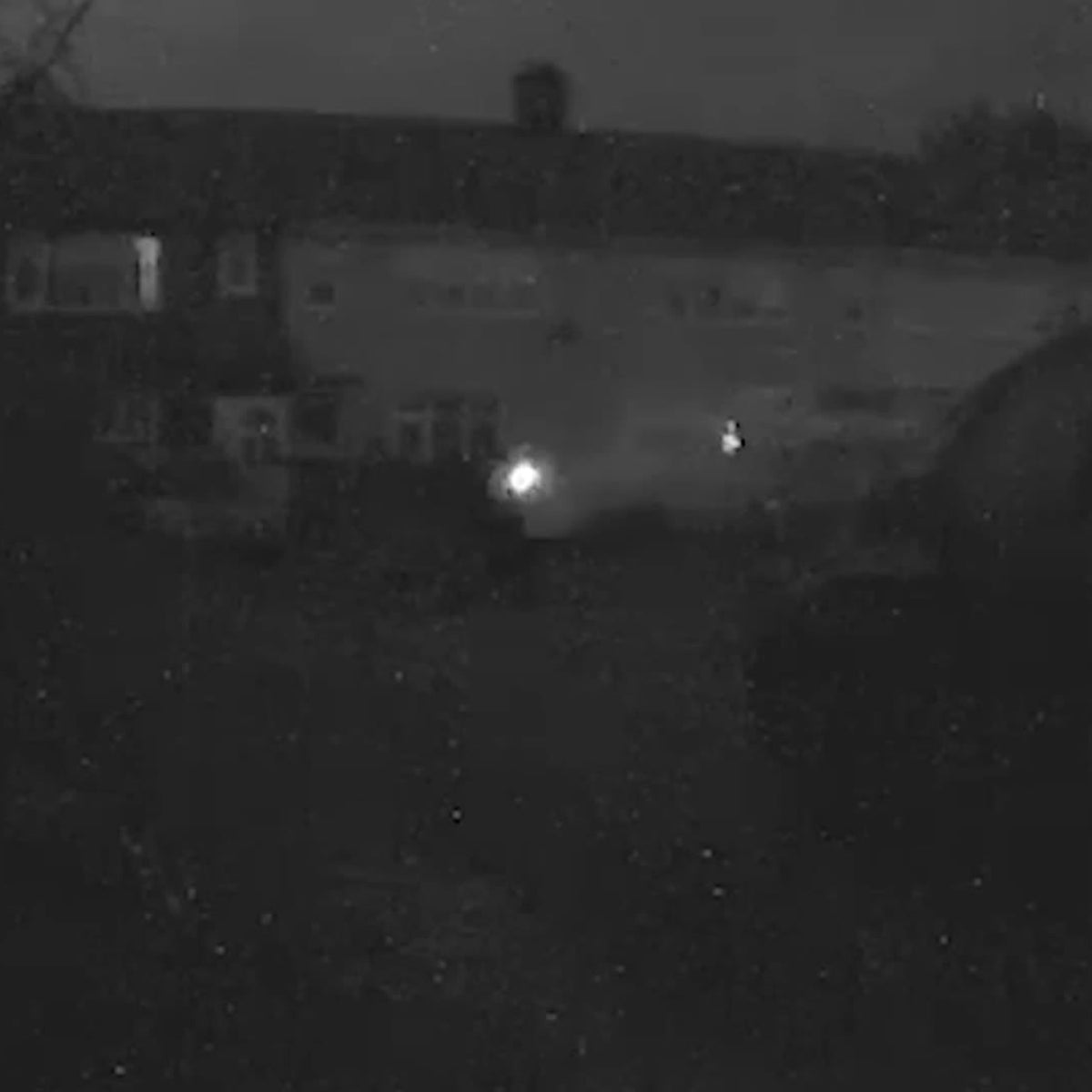The photograph is a murky, black and white image taken at night, likely with a low-quality camera. Dominated by darkness, it shows a large, two-story building in the background, characterized by multiple rectangular windows and doors. The building also features a chimney on the roof. A single, bright light source is prominently visible in the center of the photo, casting an eerie glow and creating harsh contrasts. The light is circular and resembles either a flashlight or a bright lamp aimed towards the viewer. In the foreground, indistinct black shapes and smudges might be brush or other elements that are difficult to discern. A dark-colored vehicle is parked on the right side of the building, amidst a sky that appears as a dark gray expanse.